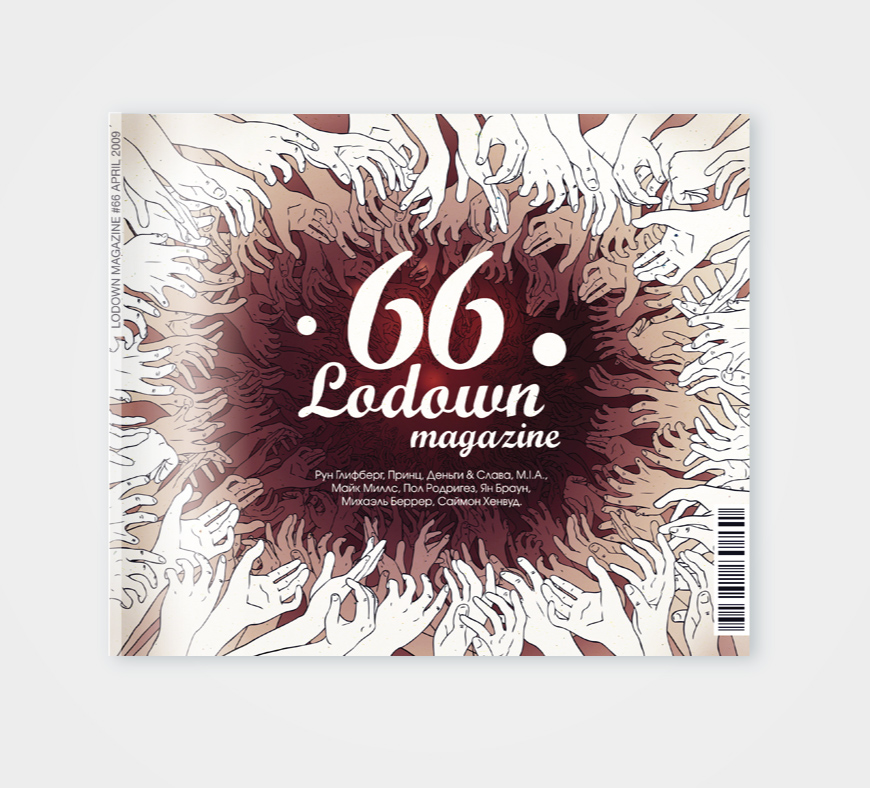The image is the cover of Lowdown Magazine, Issue No. 66, dated April 2009. The centerpiece prominently displays the title "Lowdown Magazine" and the issue number, with additional text in Russian or Cyrillic below it. Surrounding the central text, there is an intricate illustration of hands reaching towards the middle from all directions. These hands are layered and gradient, starting as white in the foreground and transitioning through shades of orange to a deep red as they recede into the background, giving a sense of depth. The hands appear to be emerging from an underworld-like abyss, suggesting a mysterious or possibly dark theme. The cover also features a barcode and an ISBN logo in the bottom right corner, adding to its authenticity as a published magazine.